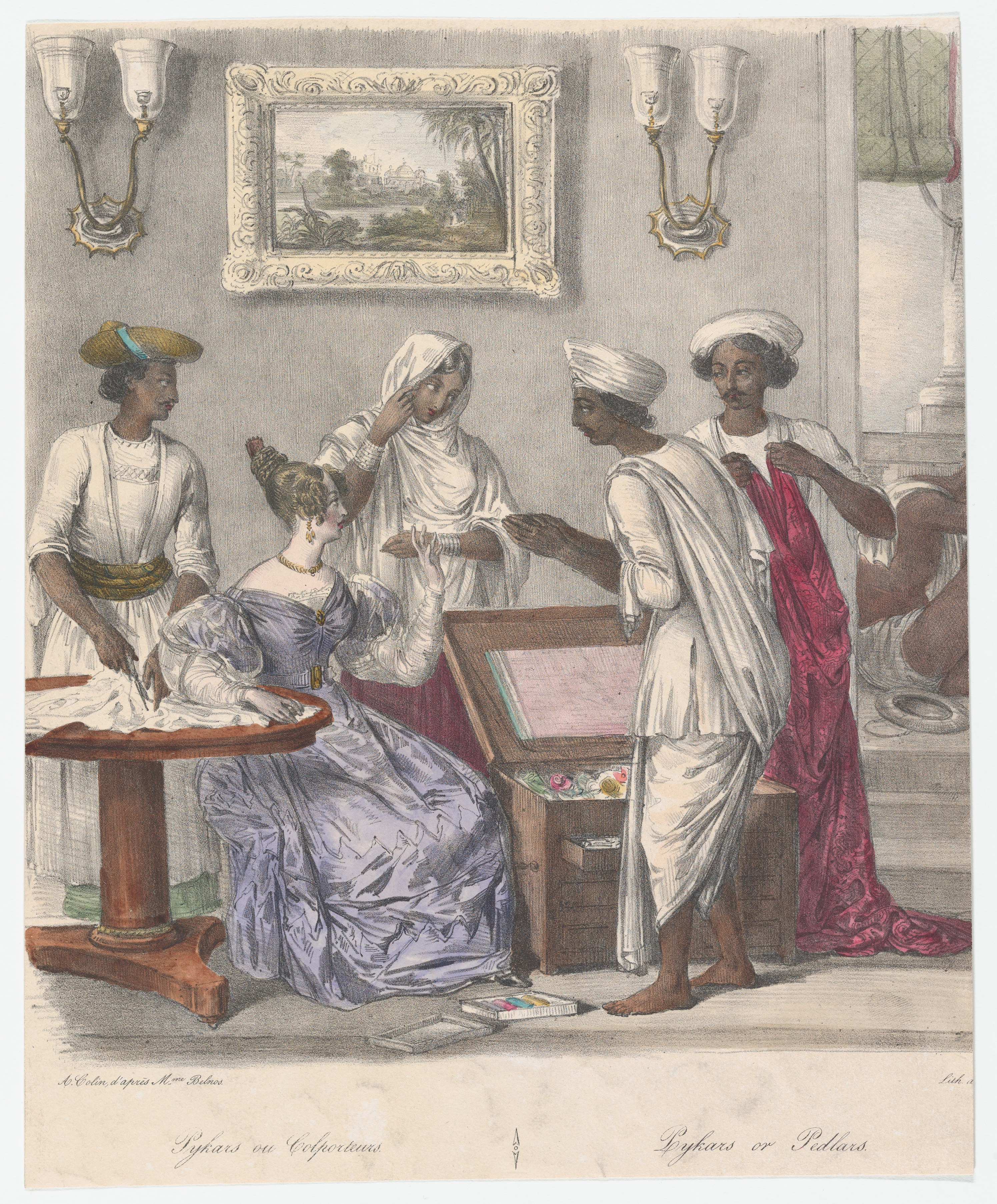This detailed painting captures an indoor scene featuring a high-class woman seated in an ornate room. She dons a full-length blue gown, her fair complexion contrasting against the darker complexions of the four standing attendants. The woman sits near a brown wooden table, and an open chest or suitcase lies at her feet. One of the male attendants, dressed in white, joins his hands respectfully in front of her, while another holds a pair of scissors, seemingly attending to her dress. Another female attendant in white holds a striking red robe up to her chest, possibly displaying it to the seated woman. The green walls serve as a backdrop, adorned with a framed painting and illuminated by light fixtures. An artist's signature marks the bottom right corner of the composition.